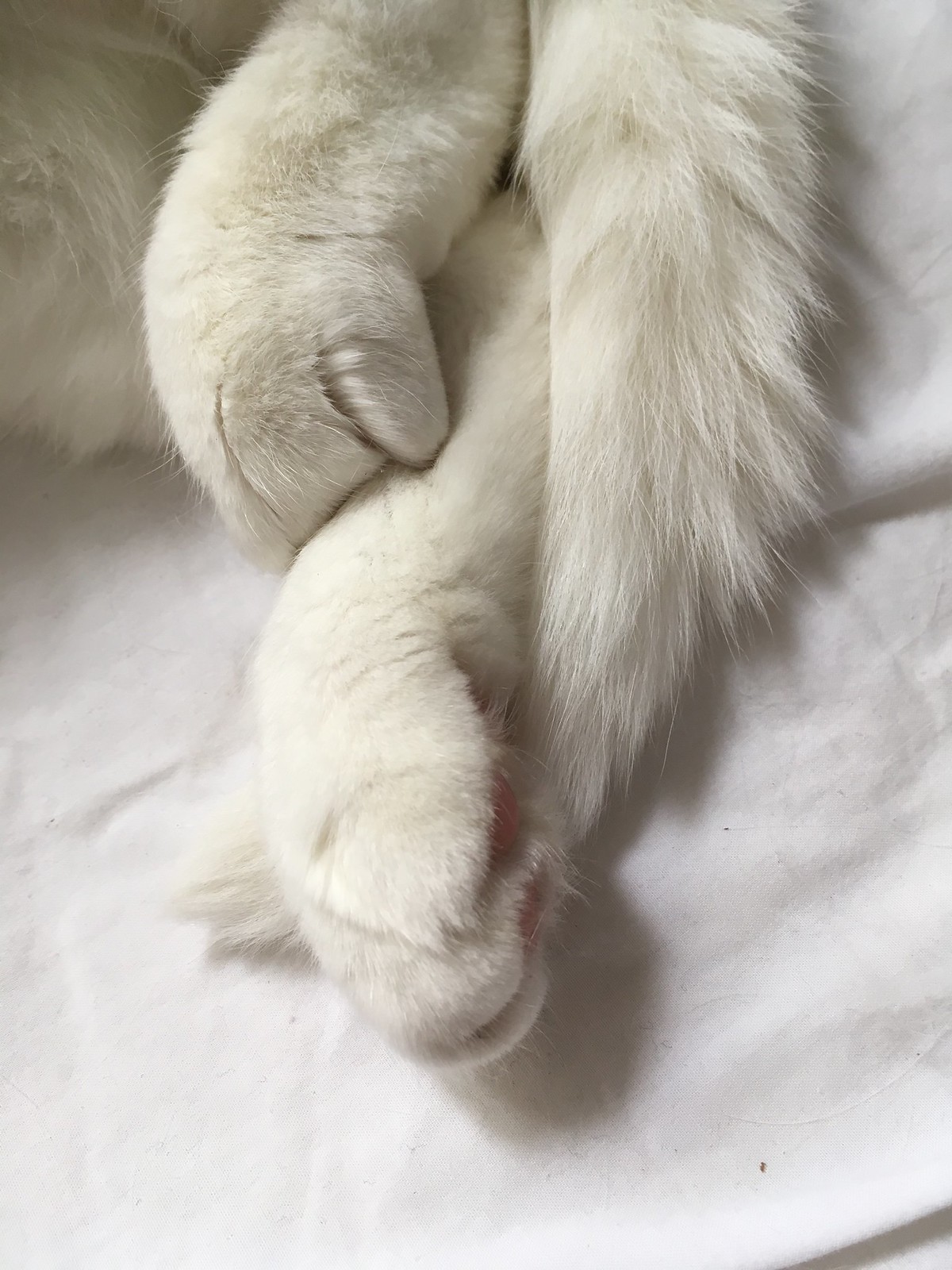In this photograph, we see a close-up of a white cat's paws and part of its tail, set against a bright white background that appears to be a bedsheet, slightly dirtied but mostly clean. The two paws and a portion of the tail enter the image from the top. The first paw extends downward and overlaps the end of the curled tail, which originates from the right side and curves to the left under the paw. The paw pads are pink, and while most of the fur is white, there are subtle gray shadows likely caused by lighting. The second paw appears curled back and resting on the other paw. Additionally, the white fur of the cat's chest is visible near the top, though the rest of the cat is cut off from the frame. The scene includes a wrinkle in the bedsheet, adding texture to the background.